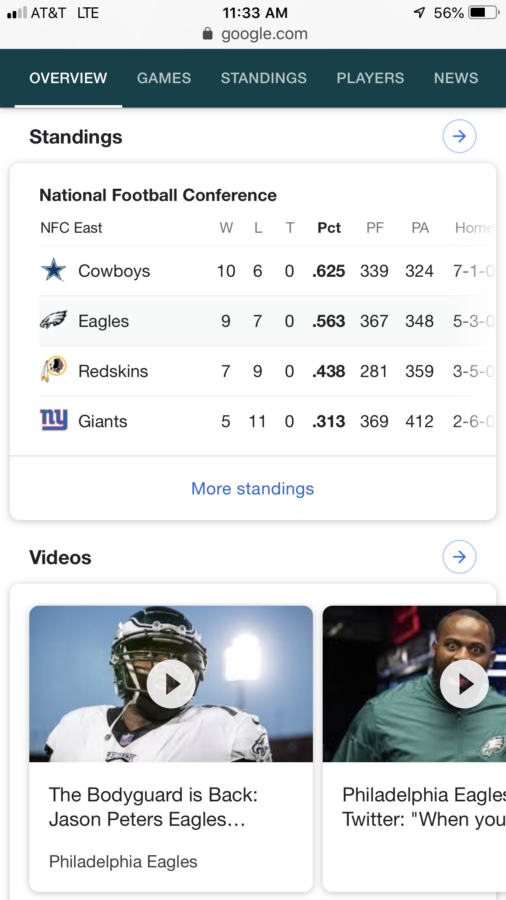The image is a screenshot of a smartphone displaying a sports app, most likely ESPN, within the Google interface. The screenshot shows the phone connected to Wi-Fi with AT&T service at two out of four signal bars. The battery level is at 56%. 

The sports app interface showcases football statistics under several tabs: Overview, Games, Standings, Players, and News. The screenshot specifically focuses on the "Standings" section under the "Overview" tab, displaying the National Football Conference (NFC) East standings. The teams listed are the Cowboys, the Eagles, the Redskins, and the Giants, in descending order based on their win-loss percentages, which are highlighted in bold. The Cowboys have the highest percentage, followed by the Eagles, the Redskins, and the Giants. There is also an option to view more standings.

At the bottom of the screenshot, there are two video previews. The first video shows a football player in full gear with the title "The Bodyguard is Back, Jason Peters, Eagles," hinting at a comeback story. The second video is partially cut off but mentions the "Philadelphia Eagles" and "Twitter," leaving the rest of the content obscured.